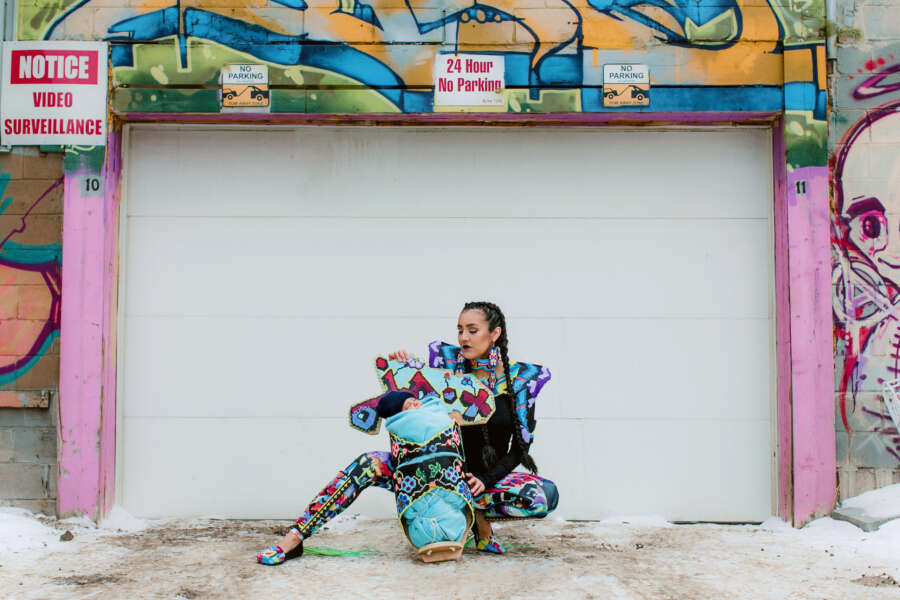In the photograph, a woman dressed in a vibrant and elaborate costume is holding up a bundled baby, similarly adorned in a matching carrier, both of which feature colorful geometric patterns reminiscent of the surrounding graffiti. The woman is standing on a flat, tan-colored concrete driveway, flanked by snow and ice. She wears a black shirt with exaggerated shoulder pads and accessorizes with black pigtails that reach her stomach, black lipstick, and earrings. The garage door behind them is white and set into a pink-painted frame. Surrounding the garage door is a diverse array of graffiti in blues, oranges, greens, and abstract patterns. Several signs are posted on the garage frame, including "Notice of Video Surveillance," "No Parking," "24-Hour No Parking," and a repeated "No Parking" sign. Numbers 10 and 11 are painted on the left and right sides of the garage door frame. The woman gazes at the baby, who is bundled in a turquoise blanket and winter hat, echoing the vivid and intricate design of their surroundings.